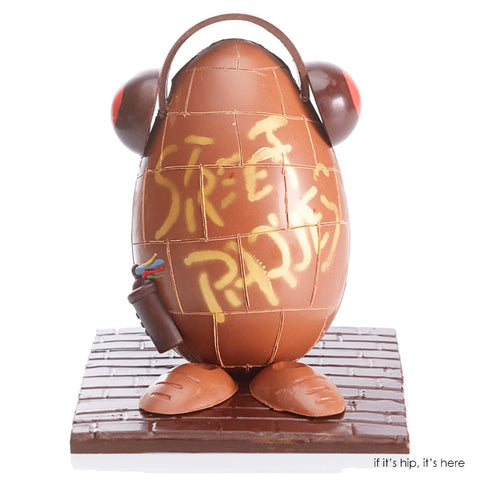The image depicts a creatively crafted chocolate egg character standing on a square base intricately carved to resemble a chocolate brick walkway, indicative of an old road. This chocolate egg, shaped perfectly round, is artistically segmented into square-like blocks with delicate lines, giving it a textured, brick-like appearance. Adorning the egg are chocolate headphones with two round orbs on either side, connected by a chocolate strap across the top. In its left hand, the character holds a chocolate spray can emitting vibrant streaks of candy colors—yellow, blue, red, and green. The egg is also wearing brown chocolate shoes. Emblazoned in gold-yellow graffiti text across its body are the words "Street Party." The image suggests it might be an invitation or advertisement for a musical street party. In the lower right-hand corner of the image, the phrase "If it's hip, it's here" is prominently featured, suggesting that attending the event aligns with being trendy or in-the-know.